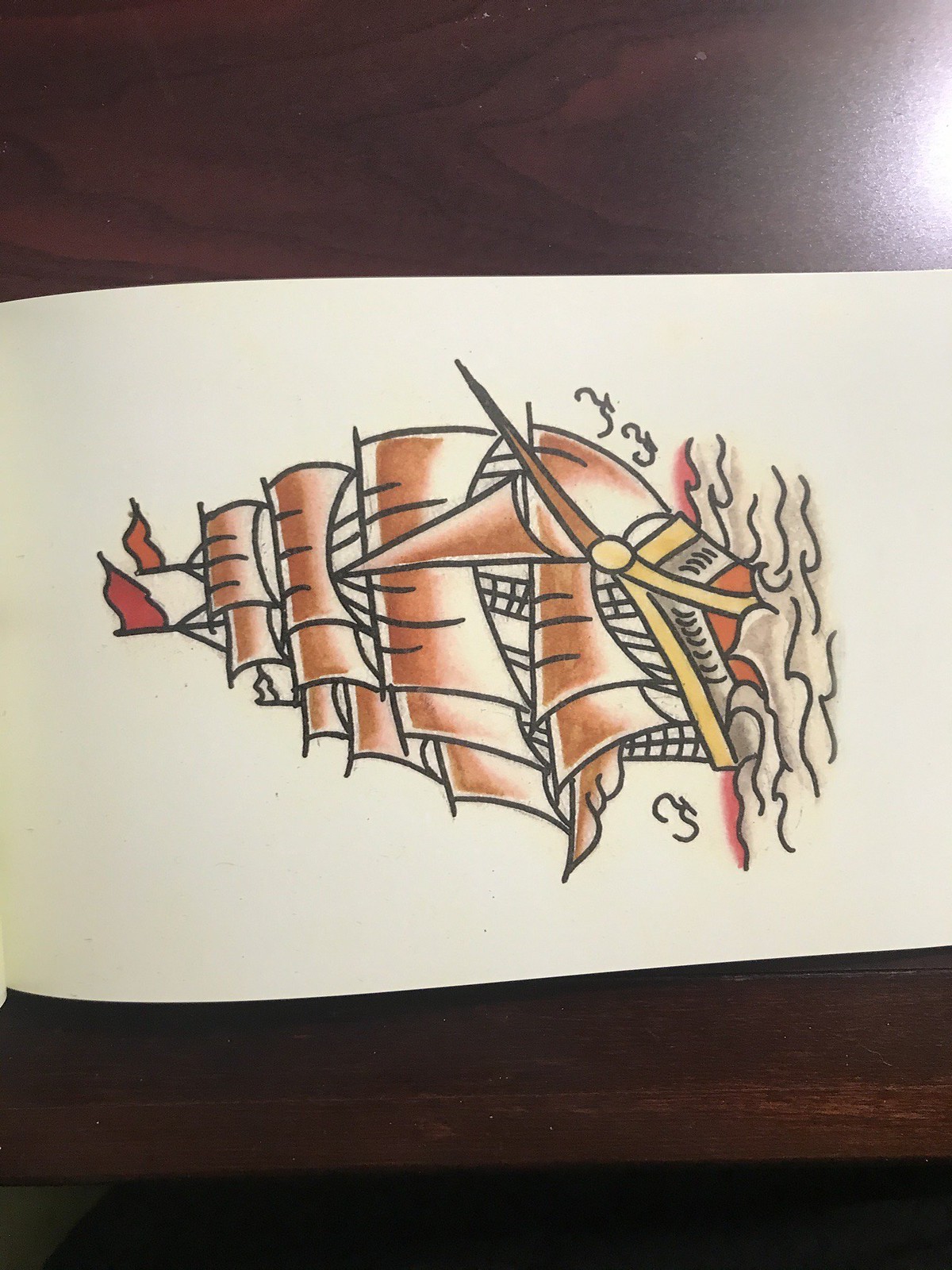A photograph captures a sketch laid on its side on a dark brown wooden tabletop. The wood grain texture is visible and there's a reflection of a bright white light in the corner, though the light source is off-camera. In the center of the table is a white piece of paper showcasing a crayon-colored and shaded drawing of an 18th-century galleon-style sailing ship. The ship's hull is predominantly red and white with gold and yellow trim details around the edges, featuring a pointy bowsprit at the front. The ship has numerous sails, shaded from brown at the top to white at the bottom, with some rust-colored accents. There's a pair of flags at the ship's top, primarily shaded in dark red and orange hues. Additionally, three simplistic, squiggly line representations of birds appear near the ship, and beneath it, gray-shaded black line waves are present, enhancing the depiction of the ship on the water.